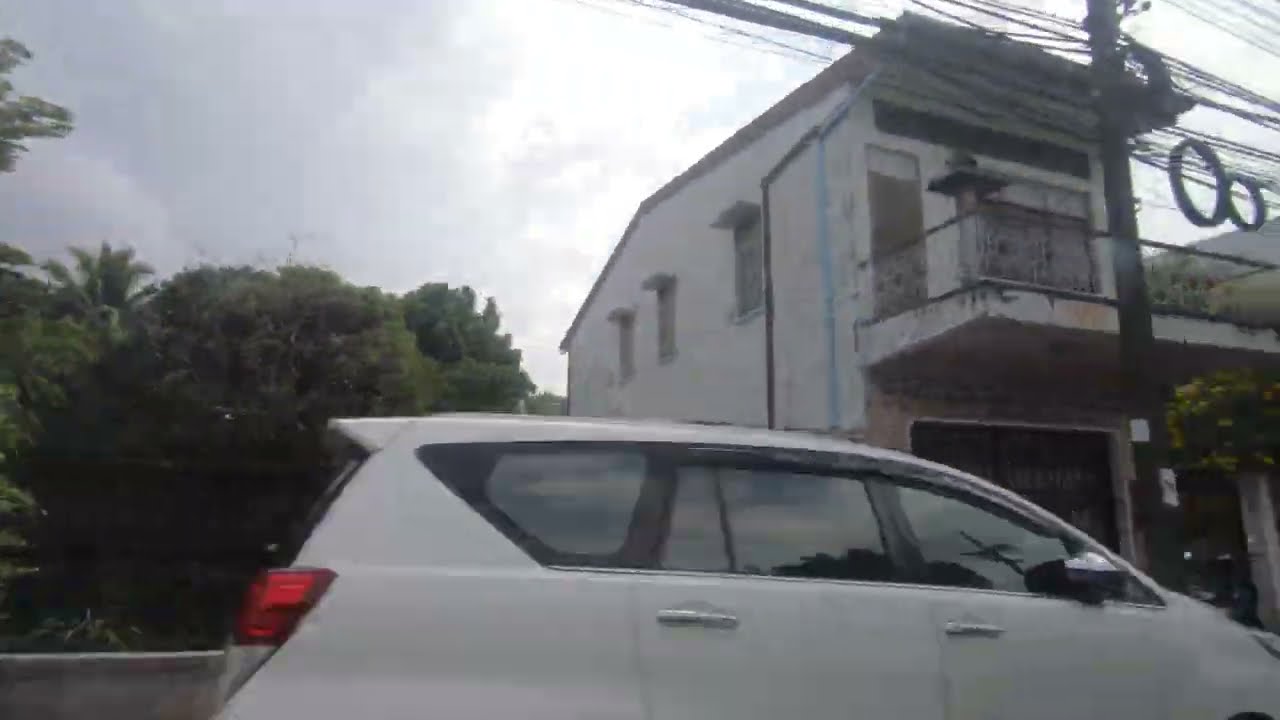The photograph captures a street-side scene dominated by a white four-door car that is parked on the side of the road. Adjacent to the car, a low cement railing separates the roadside from an entry area behind it. The sky above is dark gray and overcast, adding a somber mood to the image. On the left side of the image, various green trees, including palm trees, are visible behind the concrete barrier. To the right, there's a square rectangular white building with a patio on the second floor, overlooking a garage. This building appears somewhat narrow and is in a slightly rundown, off-white condition. In front of this building, a tall brown power line pole stands with numerous thick black utility wires extending horizontally in both directions. The overall setting suggests an urban or suburban area, potentially in an East Asian country.